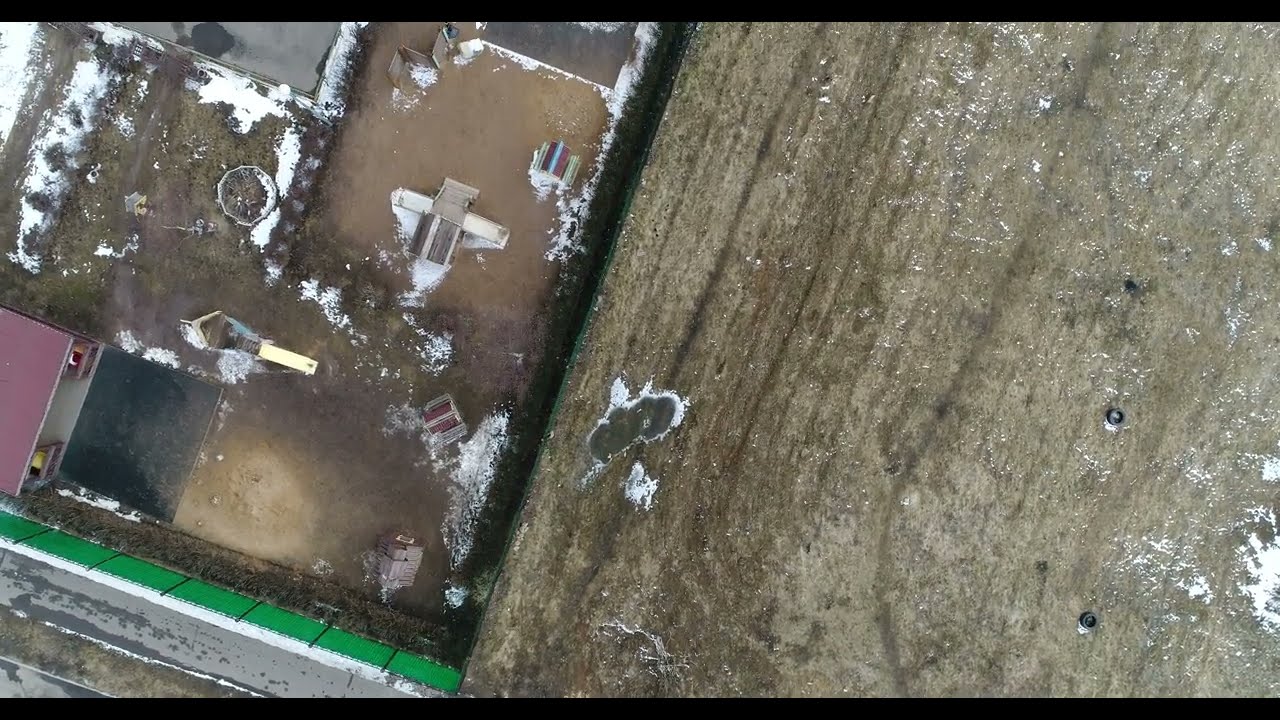This aerial color photograph, oriented in landscape perspective, captures a desolate, snow-dusted field with scattered white debris and distinct features. Prominently visible at the bottom of the image is a two-lane gray road, marked by a white broken stripe and intersected by a narrow parallel pathway. A blue sedan is present in the far right lane, adding a hint of activity to the otherwise barren scene. The field's icy, muddy expanses suggest a cold and harsh environment. In the top left corner, a partially visible building, possibly a home, further adds to the landscape's intrigue despite its indistinct form. The photograph's intent appears contemplative, perhaps taken by a landowner wishing to document their barren, wintry property.